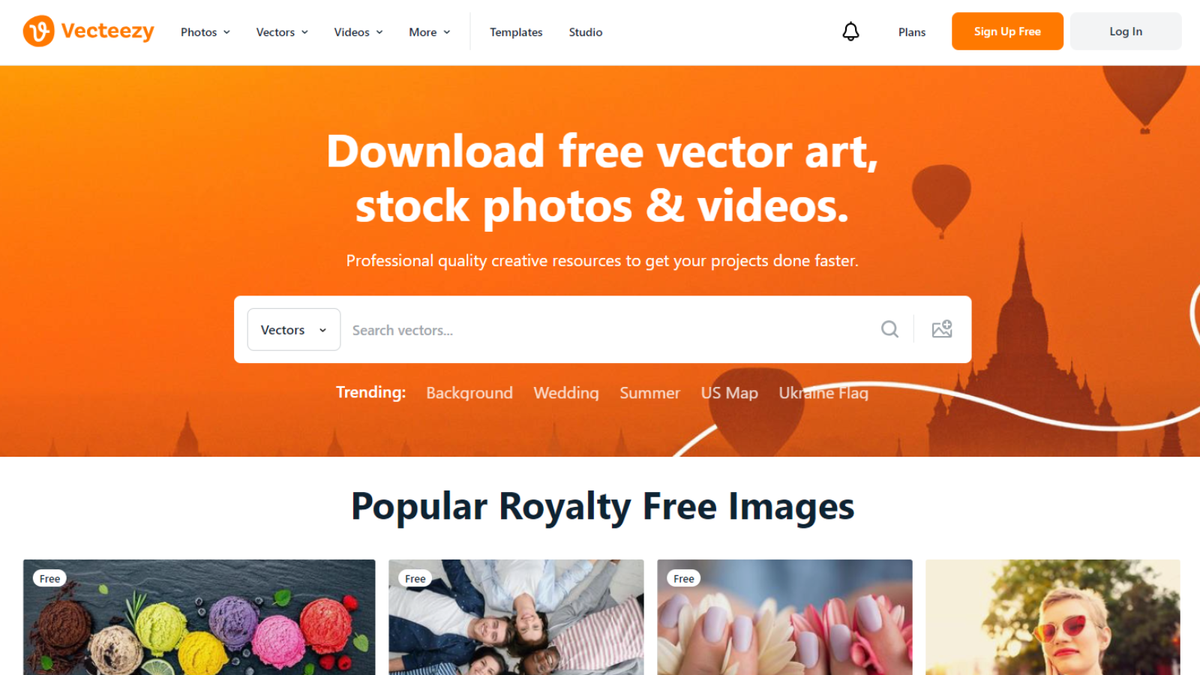The website interface of Vecteezy is showcased starting from the upper left corner. The Vecteezy logo is prominently displayed, featuring a stylized white 'V' on an orange background, with the right side of the 'V' curling upwards. Adjacent to the logo is the site name "Vecteezy."

Moving to the right, the main navigation menus are listed: "Photos," "Vectors," "Videos," and "More." Next are options for "Templates" and "Studio." Continuing along the top bar, there is an icon of a bell followed by the "Plans" section indicated with a capital 'P.' The navigation bar finishes with two buttons – an orange "Sign Up" box and a gray "Login" box.

Below the main navigation, the text "Download-free vector art, stock photos, and videos" is prominent, with a supportive tagline, "Professional quality, creative resources to get your project done now," all set within a white box. Options for vectors and search vectors are included alongside a magnifying glass icon and menu, set against an orange background.

Further down the page, there is a “Trending” section featuring popular search terms such as "background," "wedding," "summer," "US map," and "Ukraine flag."